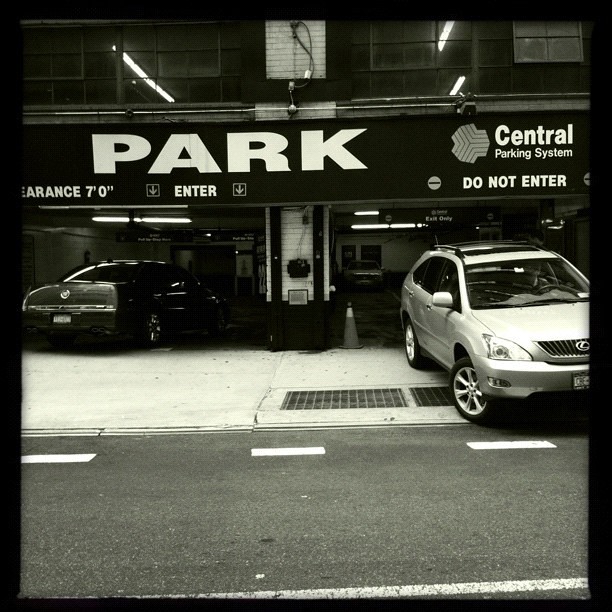This striking black-and-white photograph captures a dynamic scene of a bustling parking garage's entrance and exit. Framed by a black border, the image prominently features the facade of the building at the top. Dominating the scene is a bold black banner with large white capital letters spelling out "PARK." Directly beneath, the sign indicates a clearance of 7 feet 0 inches, with arrows pointing downward above the word "ENTER."

On the right side, the signage for "CENTRAL PARKING SYSTEM" is clearly visible, accompanied by a pair of negative symbols flanking the directive "DO NOT ENTER." Below this, a silver Lexus SUV is seen exiting the garage. In contrast, on the left side of the frame, a black car is pulling into the parking area under the guidance of the "ENTER" sign. The foreground reveals a street marked with white stripes, a sidewalk, and grates covering the sewers, while a traffic cone subtly adds to the scene. Above the parking signs, the light from inside the building filters out through multiple window panes, adding depth to the image. The photograph effectively captures the rhythm and flow of vehicles navigating the parking system.